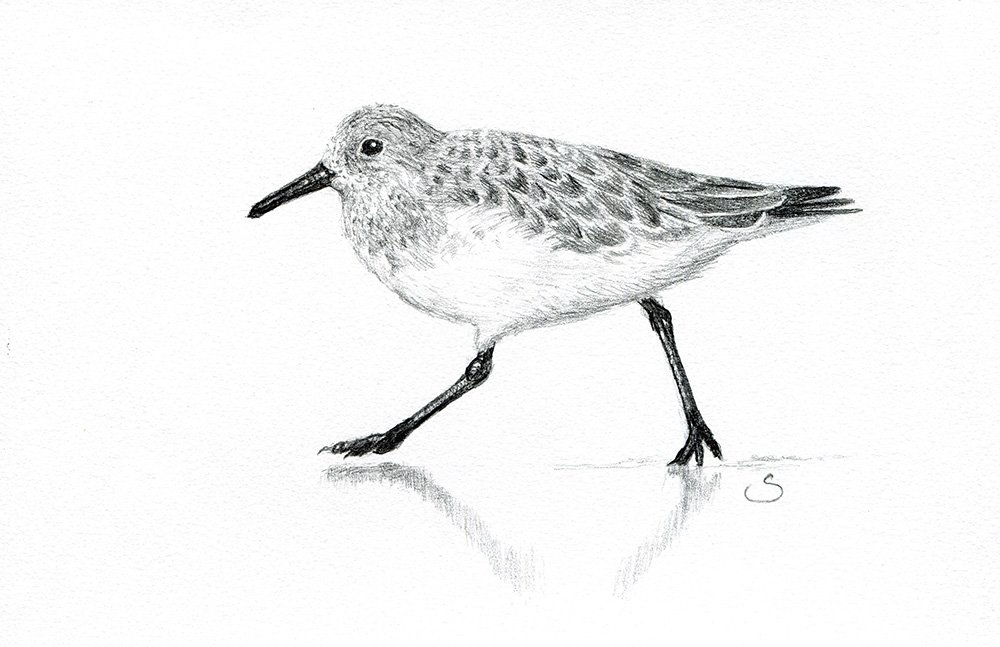The image is a black and white pen and ink drawing of a small bird. It's designed with intricate detailing, featuring a white chest and gradually darkening feathers towards the back, culminating in a black tail. The bird has a prominent, long black beak and equally long black legs, which are outstretched as it walks; its left leg is forward while its right leg is extended back. The bird's eye is black, and it has gray scaling on its head and wings. There is a subtle reflection beneath its legs, indicating the surface it walks on, which is a light gray hue against a plain, matte white background. The image is horizontal, and a stylized, cursive letter "S" appears on the right side near the back leg of the bird.